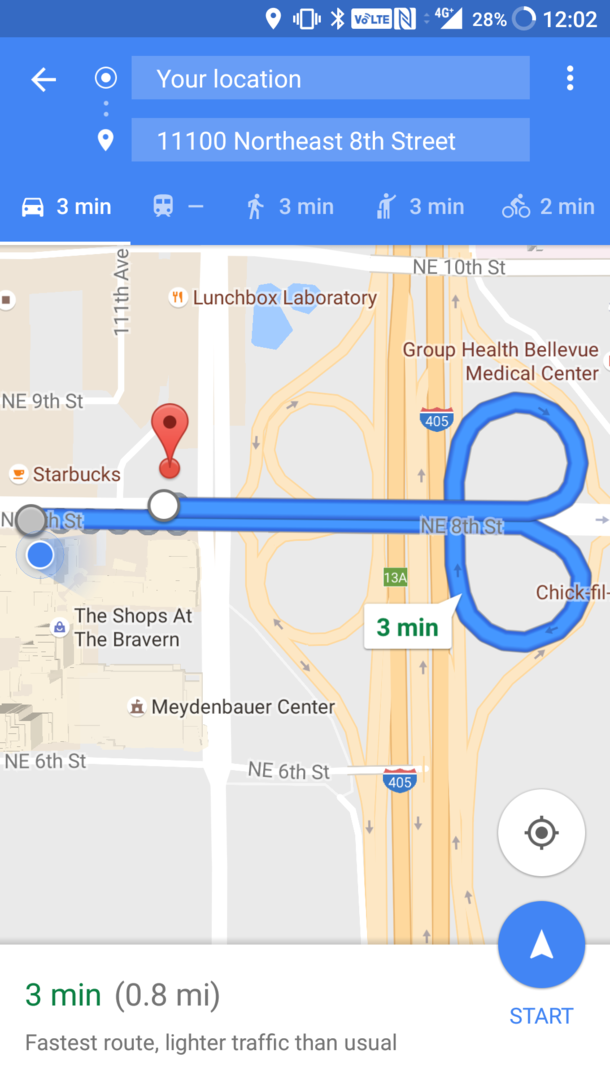This image, captured on a smartphone, displays a digital map interface. At the top of the screen, the phone's status bar is visible, featuring a dark blue border where a vibrating phone icon is shown, indicating 4G connectivity. The battery level is at 28%, and the time displayed is 12:02. Below this, there is a slightly lighter blue bar with an arrow pointing left and two sections. The top section reads "Your Location," and the bottom section indicates "11100 Northeast 8th Street."

Beneath this, there are multiple transportation options, including car, bus, walking, biking, and another option showing a person holding a suitcase, possibly indicating public transit. The estimated travel times are three minutes by car, two minutes by bike, and three minutes on foot. A blue line runs down the center of the map, forming two loops at the ends, with a red dropped pin marking the destination. A label points to one of the loops, indicating that it is a three-minute journey.

Various landmarks are marked on the map, including a "Lunchbox Laboratory" at the top with a fork and knife icon, "Starbucks" on the far left, and "Chick-fil-A" on the far right. Centrally located are "The Shops at Bravern" and "Mabowern Center."

This detailed caption provides a comprehensive description of the map and its features, making it clear and informative.